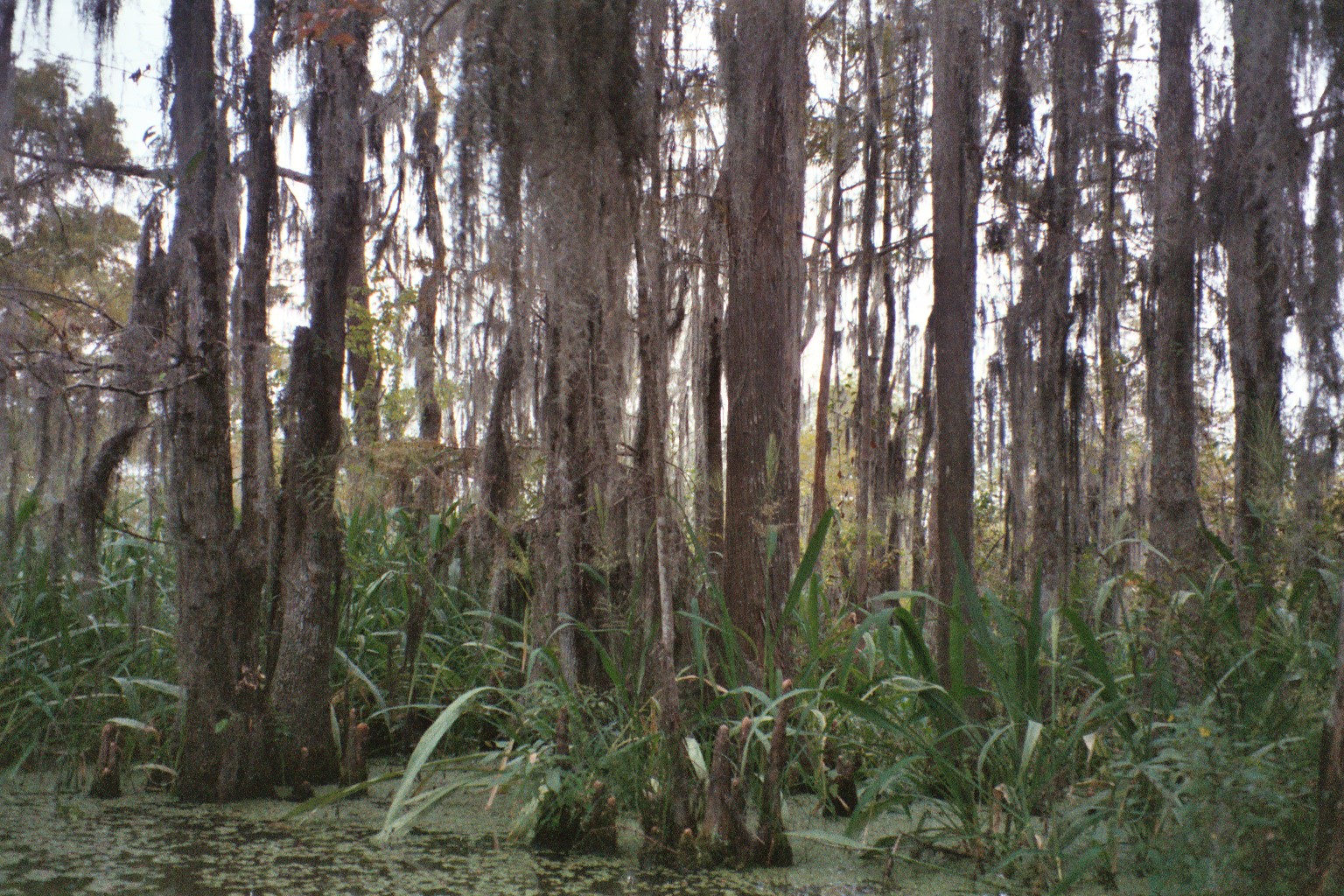This colored photograph captures an outdoor scene during the daytime featuring a scraggly, unkempt forest, likely situated within a Floridian swamp. The tall, slender trees exhibit ashy, dark brown trunks, many of which are obscured by hanging vines, characteristic of the region's swampy areas. Sparse blue sky peeks through the thick canopy of the forest. The backdrop reveals a swampy terrain, with visible swamp water covered in scum, contributing to an overall muggy atmosphere. The ground is carpeted with green moss and interspersed with tall, weedy grasses and greenish shrubs. While most trees appear bare or wilting, a large bush commands attention in the bottom right corner, and a tree with abundant leaves stands out towards the far left. No animals or people are present, emphasizing the untouched, natural state of this swampy forest.